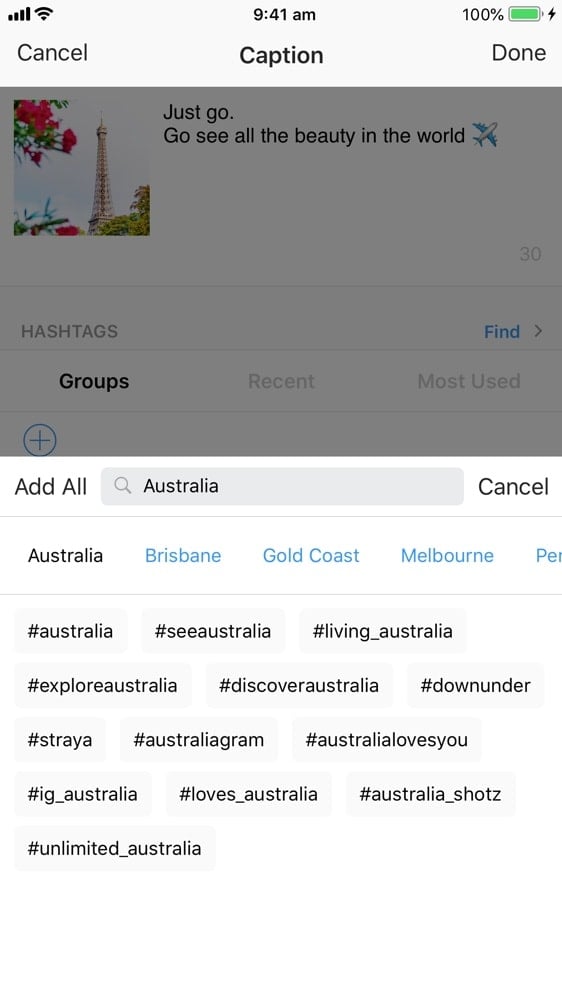A screenshot of a smartphone screen is captured, detailing various user interface elements. 

At the top, the status bar displays a black Wi-Fi symbol indicating full signal strength, the time reading "9:41 a.m.", and a green battery icon showing 100% charge.

Below, the screen shows an app interface featuring a gray box containing an image. The image depicts a tall, thin gold structure surrounded by vibrant pink and green flowers. Below the image, a motivational quote in black font reads, "Just go. Go see all the beauty in the world," followed by a white and blue airplane icon.

The app interface includes numerous interactive elements. A gray search box labeled "Australia" features a magnifying glass icon and a "Cancel" option in black. Below, the word "Australia" appears in black, followed by "Brisbane," "Gold Coast," and "Melbourne" in blue.

A collection of hashtags, each enclosed in gray boxes and written in black text, populate the lower section of the screen. These hashtags include:
- #Australia
- #SeeAustralia
- #Living_Australia
- #ExploreAustralia
- #DiscoverAustralia
- #DownUnder
- #Strya
- #AustraliaGram
- #AustraliaLovesYou
- #IG_Australia
- #Loves_Australia
- #Australia_Shots
- #Unlimited_Australia

The overall image is crisp and clear, offering excellent readability and detailed visual information.